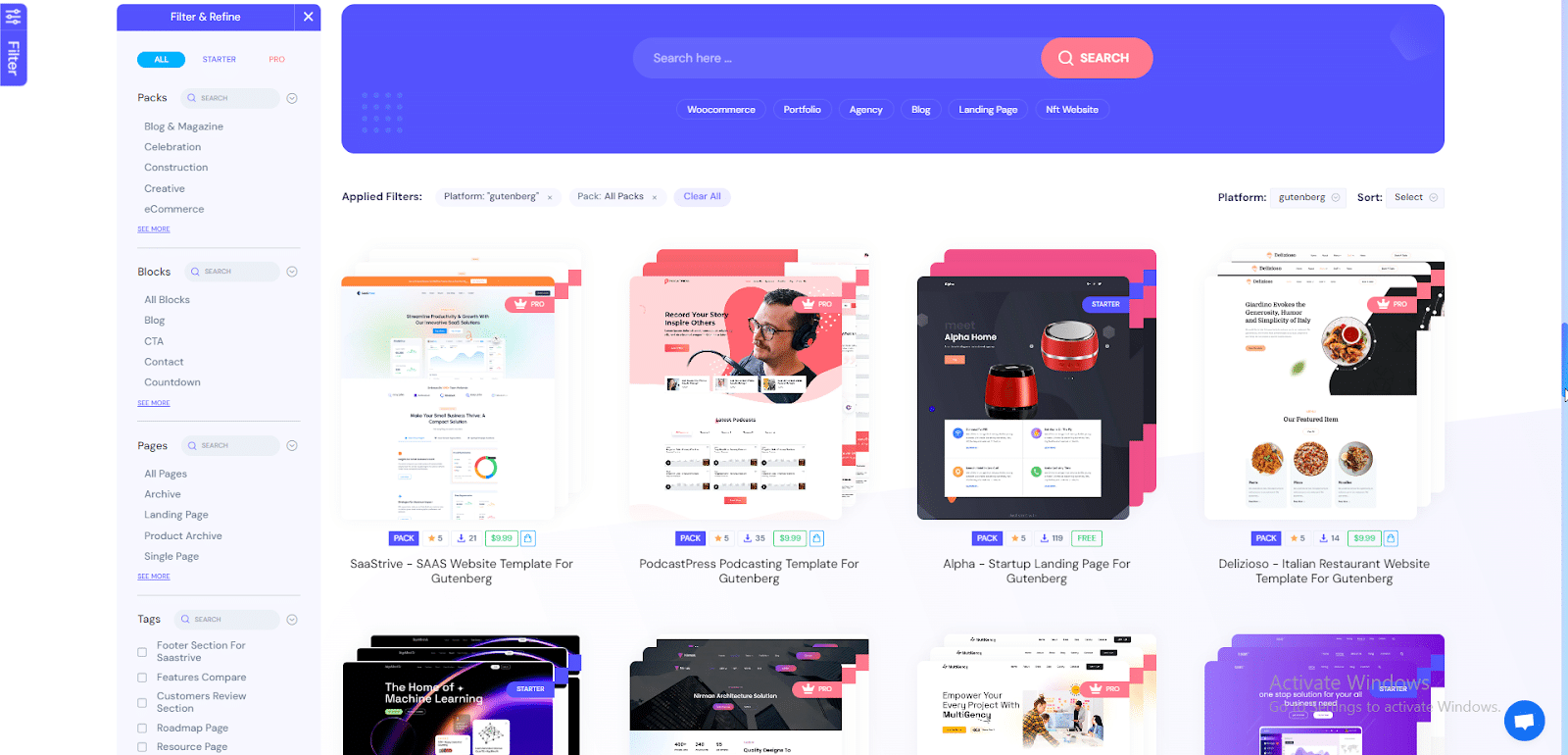This image showcases a detailed screenshot of a website, focusing on its layout and navigation elements. On the far left, there is a vertical filter menu represented by a small button labeled "Filter." Moving further to the right, the vertical menu includes several sections, each designated with a white font on a purple background. The menu categories are as follows: "All," "Starter," "Buttons," "Pack," "Block," "Pages," and "Tags." 

Above the main content area, there is a prominent banner featuring a search bar, accompanied by a search button for easy navigation. Below the banner, the content area displays two rows of website templates. Each row contains four individual templates, complete with their respective prices prominently displayed. The layout and design elements suggest a user-friendly interface aimed at facilitating the selection and purchase of website templates.